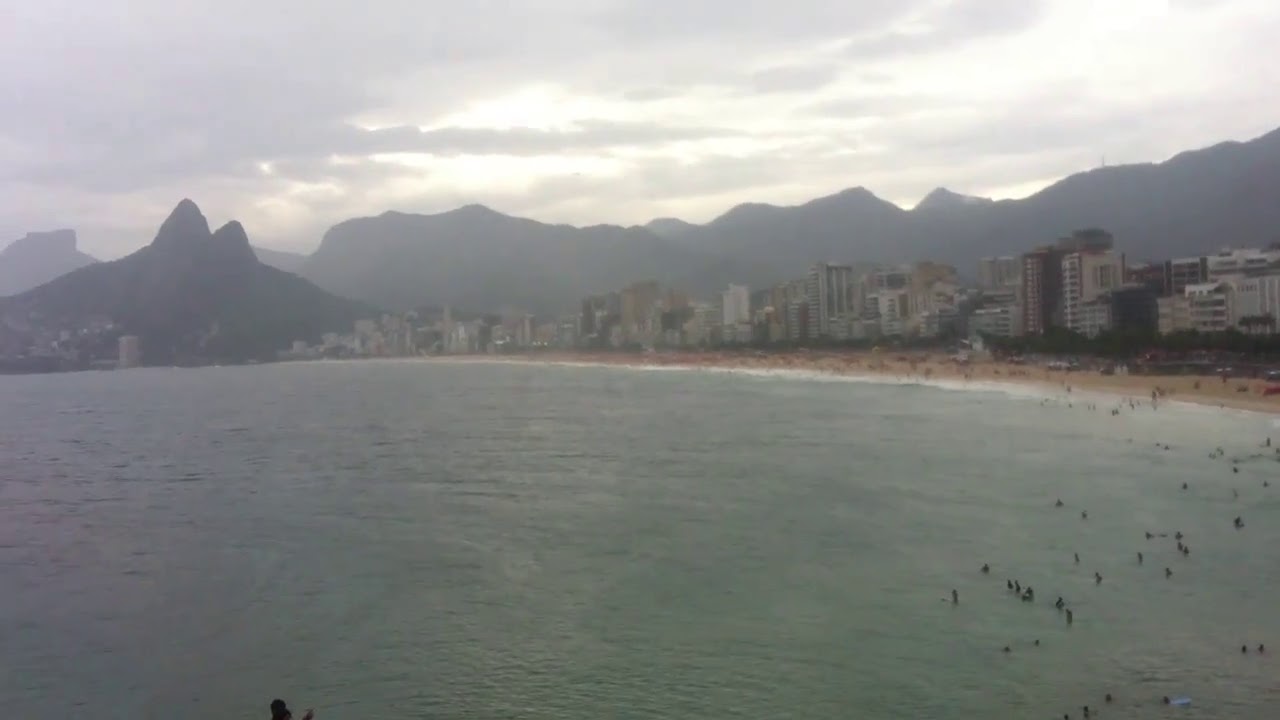The image depicts a coastal scene featuring an expansive harbor with a curved beachline extending to the horizon. The ominous gray water is dotted with swimmers, particularly concentrated on the right side. At the center, the sandy beach is populated with numerous people, though individual details are indistinguishable due to the distance. The beach is surrounded by shrubbery and transitions into a cityscape characterized by high-rise buildings, including tenements and hotels, with many featuring balconies. The cityscape sits against a backdrop of dark, gray hills and mountainous outcrops, some towering approximately 1,000 feet. The sky above is a blend of gray and white clouds, with brighter white skies emerging behind the towering hills, enhancing the dramatic atmosphere. The scene is imbued with a palette of gray, white, brown, tan, green, blue, orange, and red, indicating various elements in this middle-of-the-day, outdoor setting.